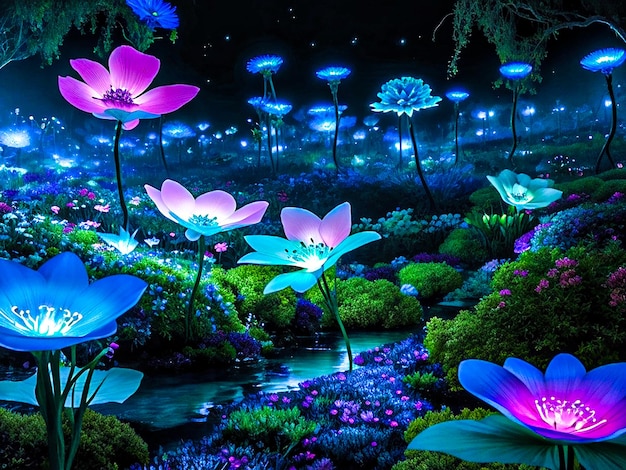This stunning color illustration depicts a magical, glowing garden under a black, star-filled night sky. A serene stream meanders through the middle, flanked by various plants. In the foreground, luminous water lilies with bright, glowing centers float gracefully, with flowers in shades of blue and purple, some sporting both lavender and turquoise leaves. Surrounding the water are mounding plants with cascading blue flowers. Lower green plants and blue-green flora adorned with purple and pink blooms add to the enchantment. The background stretches to the horizon with fields of glowing flowers, including aster or daisy-shaped ones with blue petals and white, radiant centers. A large, blue carnation-shaped flower stands prominently, while drooping tree branches frame the scene from the top corners. The entire landscape emanates a serene, fantasy-like atmosphere, with the glow of the flowers resembling fireflies in all shades of blue and purple. A faint image of a butterfly, or perhaps another flower, can be seen in the bottom left, enhancing the overall mystical allure.